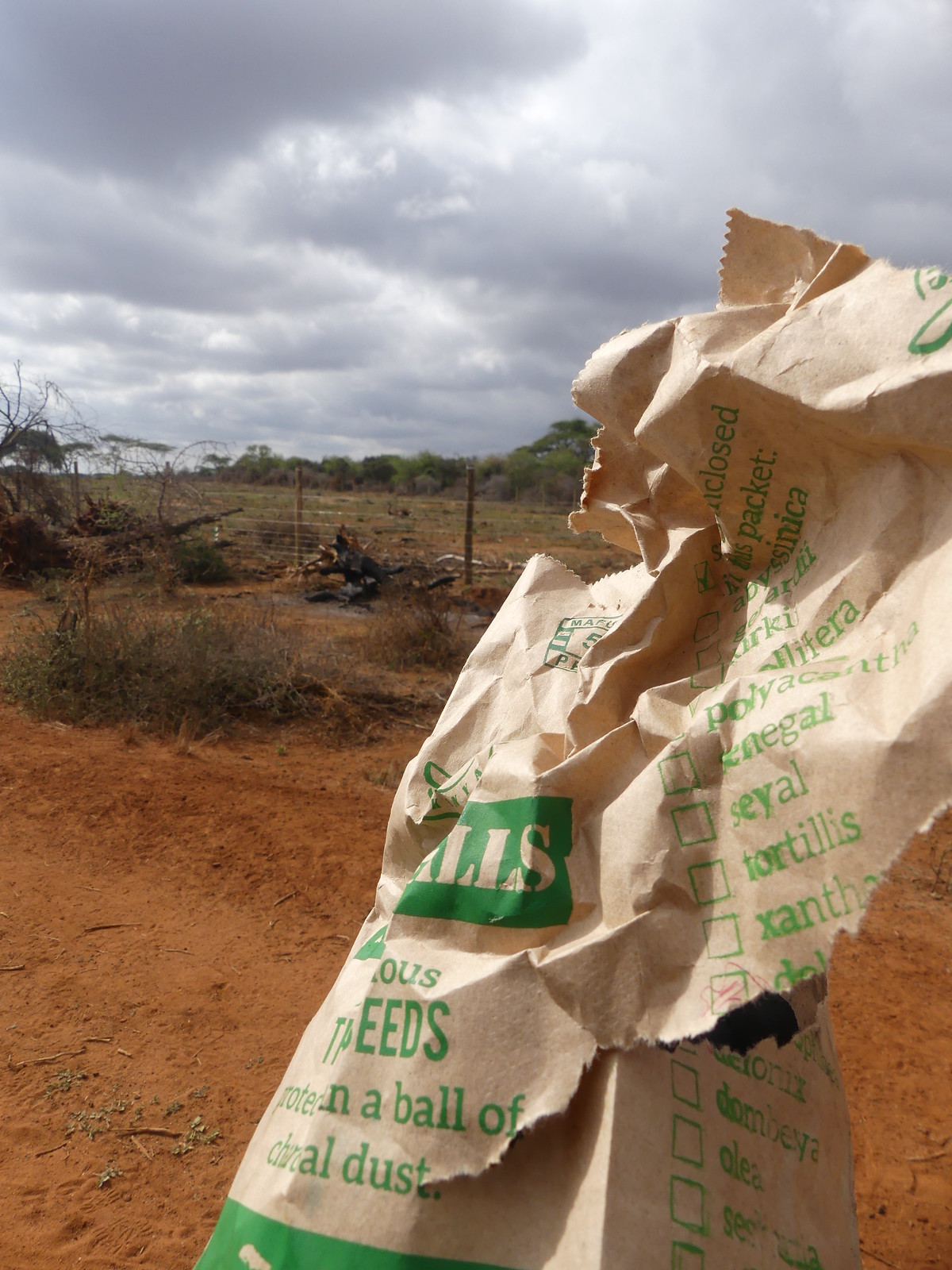A vertical photograph depicts a rural farmland under a gray, cloudy sky. At the top of the image, dense clouds blanket the sky, setting a somber tone. The horizon cuts through the upper section of the photograph, just below the clouds. Centered and stretching horizontally is a rustic wooden fence, defining the boundary between the cultivated land and the foreground.

In the bottom right corner, a torn piece of paper or a ripped up paper bag lies discarded on a dirt road or open dirt area. The paper features text, though words are partially obscured and challenging to read; hints of "tortillas," "dust," and "xanthan" can be faintly discerned.

The landscape is a mix of green fields, contrasting with the brownish dirt road and fence, while the sky remains a consistent gray. Scattered colors include shades of white, beige, and black, adding to the neutral and earthy palette typical of such rural settings. The entire scene captures an outdoor, daytime moment in a remote farming area on a cloudy day.